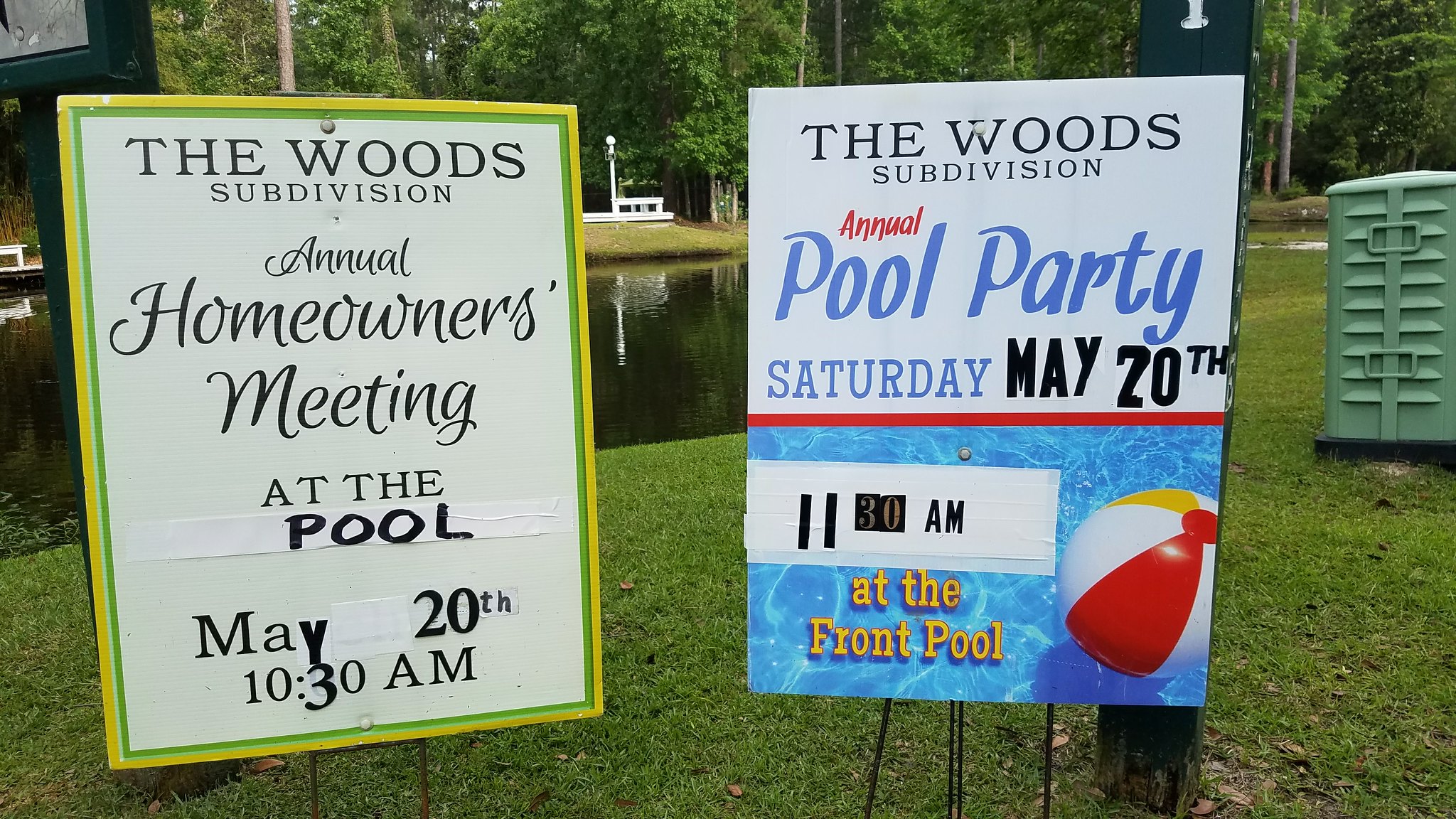The image features two informative signs positioned outside on a grassy field. Both signs stand on tripods, enhancing their visibility. Behind the signs, a serene body of water can be seen, bordered by lush green trees.

On the left, the sign has a white background framed by a narrow green and yellow border. The text in black reads: "The Woods Subdivision Annual Homeowners Meeting at the Pool, May 20th, 10:30 AM."

The sign on the right has a white background on its upper half. It announces in black text: "The Woods Subdivision Annual Pool Party, Saturday, May 20th." This text is interrupted by a red line that extends across the flyer. Below the red line, there is an image featuring a beach ball floating in blue pool water, with the time "11:30 AM" written in black, accompanied by the words "at the front pool" in yellow.

A metallic green contraption appears to the right of the signs, blending into the verdant backdrop of grass, pond, and trees, further emphasizing the natural outdoor setting.